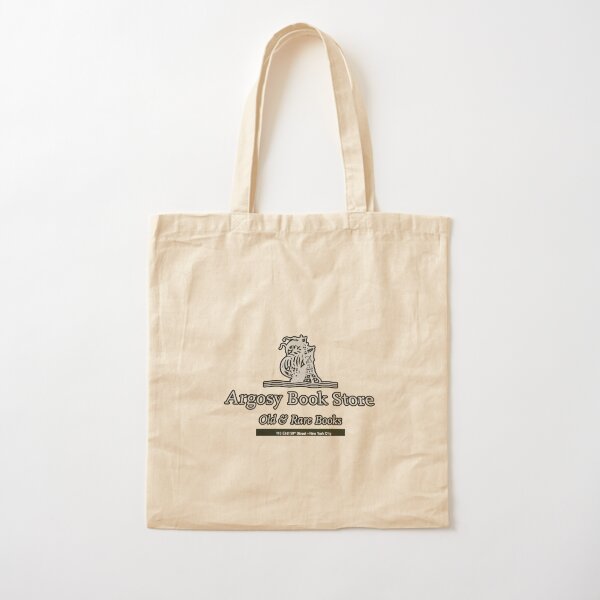The image showcases a close-up of a tan, wrinkly fabric bag, possibly made of canvas, set against a white backdrop. The bag features two sturdy, ample straps that suggest it could be carried by hand or draped over the shoulder. On the front of the bag, there is a somewhat abstract and statue-like design whose details are not entirely clear due to its indistinct quality. Below this design, the bag prominently displays the text "Argosy Bookstore" followed by the tagline "Old and Rare Books." Further down, there's a black block of text that is too small to be legible, possibly indicating the bookstore's location or address. The overall image is brightly lit, clear, and sharply focused, with nothing else in the frame to distract from the bag itself.